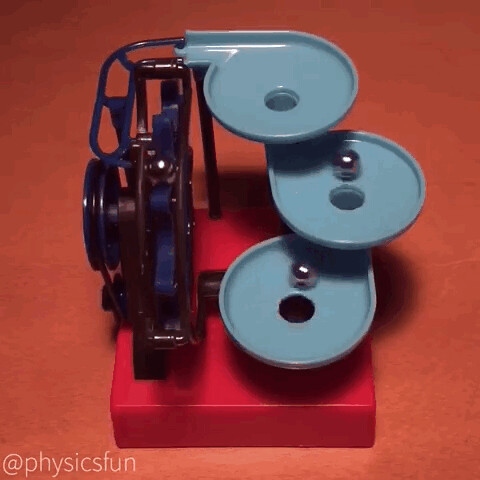The image depicts a toy-like piece of machinery set against a vibrant orange background. This vertical rectangular toy features a red base and a navy conveyor belt system that elevates silver metal balls, similar to a roller coaster. The conveyor mechanism includes a brown steel structure and a blue sprocket wheel on the left side. As the wheel rotates, it lifts the balls to a series of descending blue circular trays, each with a single hole. The balls sequentially drop from one tray to the next, ultimately reaching the bottom. The piece is a playful illustration of a marble run or physics toy, and in the lower left corner, it displays the white text "@physicsfun," signifying its connection to educational entertainment.